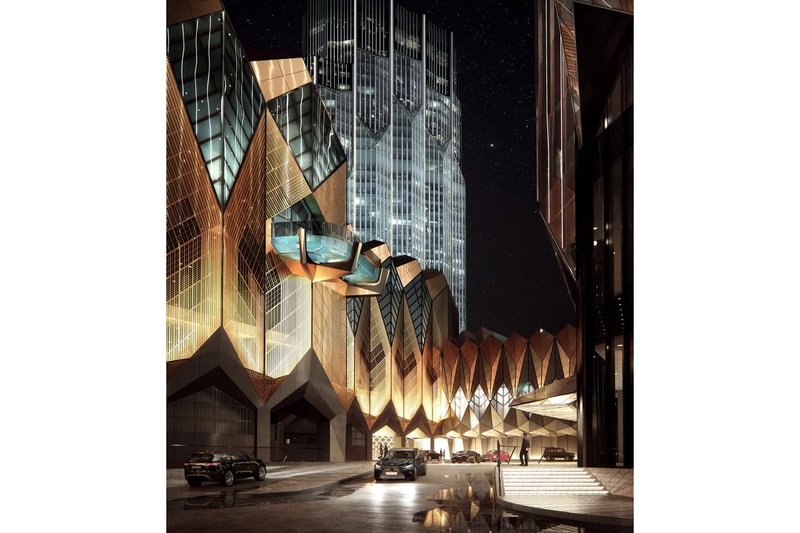In this night-time image of a futuristic city that could easily be mistaken for Dubai, a glitzy and very modern building stands as the focal point, bathed in a golden light that accentuates its geometric and jagged edges. The building features a grand, illuminated awning or arrival deck where a few cars are seen making drop-offs or pick-ups, their types indiscernible due to the distance. Large structures with diamond-like patterns and leaf-like shapes frame the awning, adding to the building's captivating design. To the left, a series of glass towers rise into the starry sky, their facades varying in shades of dark, light, and blue glass. On the edge of the street, which curves away to the right, a man stands near what appears to be a jeep or SUV, gazing at the architectural marvel. The scene is set against a dark, starry background, enhancing the dramatic and somewhat dystopian atmosphere of the cityscape.